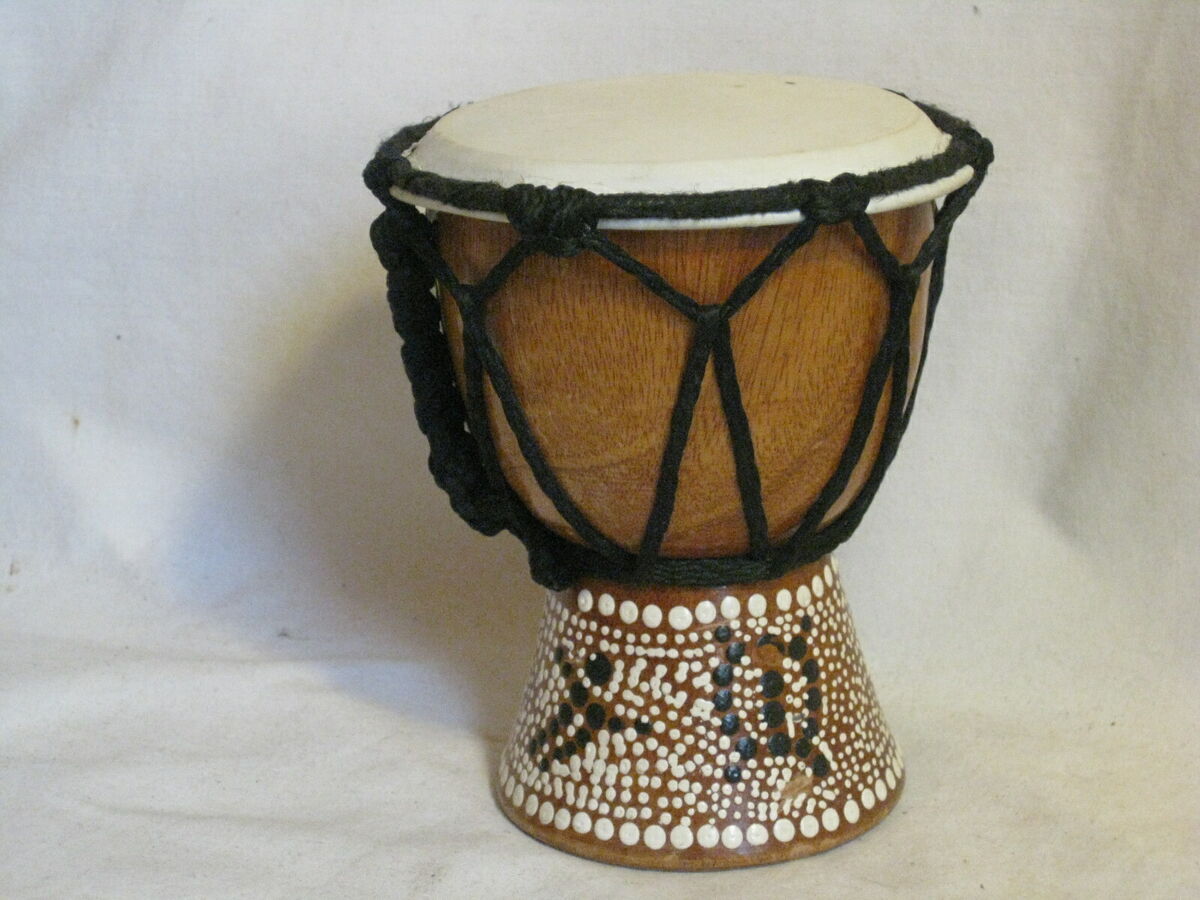This photograph features a tall, brown drum shaped like an upside-down bell or flower pot, set against a white background. The drum's distinctive design includes a white top and is adorned with a series of beads and intricate rope work. The body of the drum is wrapped in black braided rope, which also loops around the top, possibly to secure the drumhead. 

Decorative elements include larger white beads at both the top and base, interspersed with smaller white beads forming patterns. Notably, the drum features two symbolic designs made from black beads: one resembles a person with a defined head, arms, and legs, and the other seems to depict a turtle with four brown beads representing legs, a rounded back, and a central black line. The drum is set against a pristine white background that extends to the wall behind it.